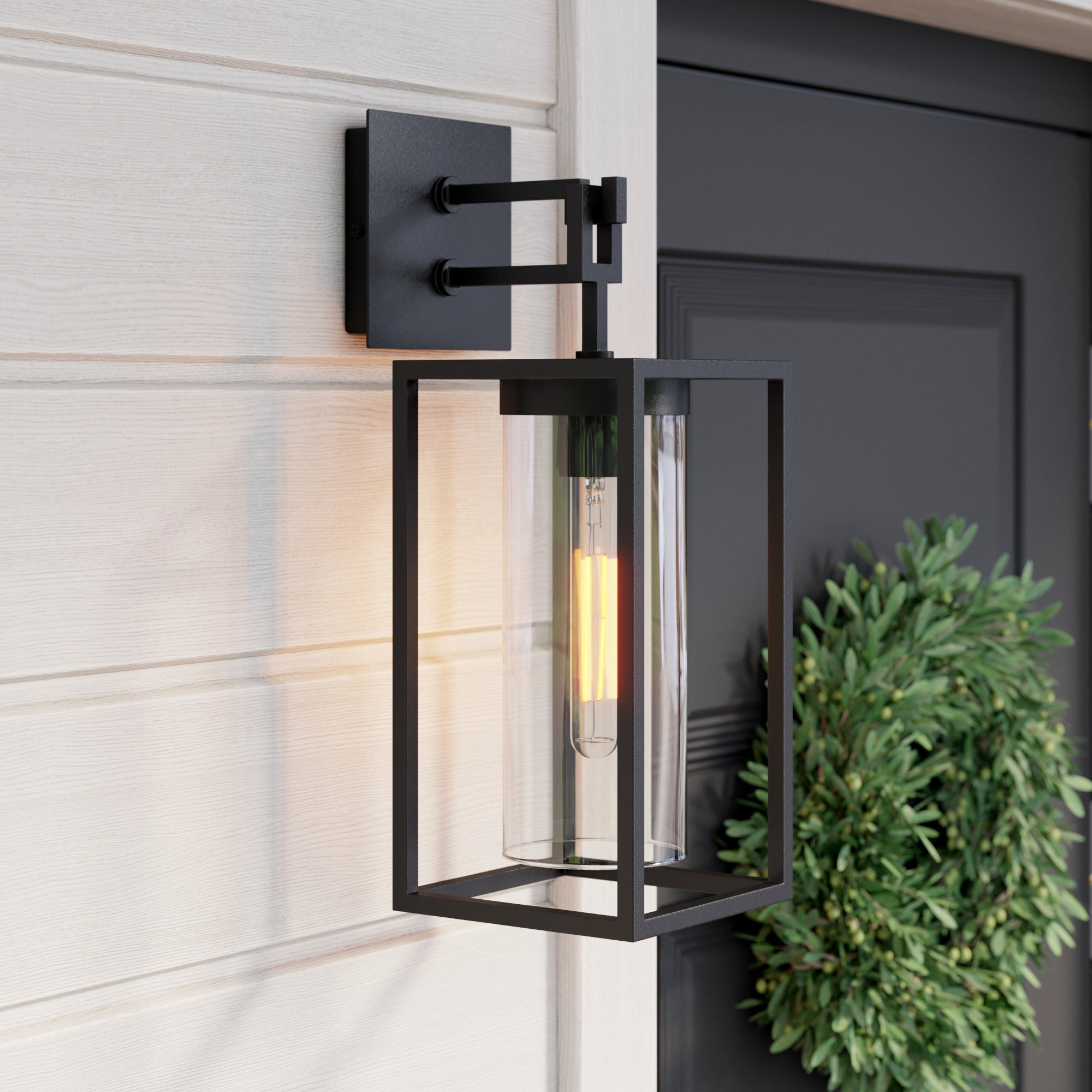The image depicts the exterior of a home, centered around a modern matte black rectangular lighting fixture attached to the side of the building. This fixture is supported by a black panel with two horizontal rods that hook vertically to hold the lantern. The lantern itself is a metal-framed rectangle that encloses a cylindrical glass cover with a slim, elongated light bulb inside. The light is mounted on a gray wall that complements the home's primary colors, which include grayish beige and black accents. Adjacent to the light is the home's front door, which is black and adorned with a green wreath, suggesting a holiday season, potentially Christmas or New Year's. There are no people or text in the image, giving the scene a staged, pristine look that highlights the home's modern aesthetic.